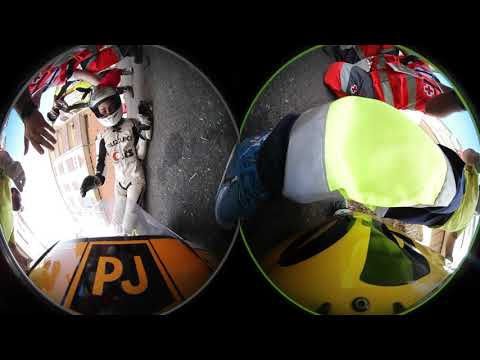The image features a heavily distorted, fisheye-lens view from a helmet cam, divided into two circular sections against a solid black background. The scene appears to capture a motorcycle accident involving a racer. In the left circle, the main focal point, a person—possibly a female motorcycle racer—is lying on the ground in a white one-piece racing suit trimmed with black and adorned with sponsor logos. She is wearing a white helmet, and a hand is reaching towards her, suggesting immediate assistance. The front of an orange motorcycle with 'PJ' in orange letters is visible, along with a small windshield. Several individuals, including at least two in yellow and one in red emergency response attire, are seen rushing to her aid.

The right circular image, dominated by the distorted perspective, shows the scene from the opposite side. Here, the knee of a person kneeling towards the racer takes up most of the frame. A yellow vehicle and a red medic bag marked with a white cross are visible, indicating emergency medical response. Additional details include a person in blue tennis shoes and elements in red and gray with emergency cross signs. The overall composition captures the urgency and chaos of the accident scene with significant emphasis on rescue efforts.